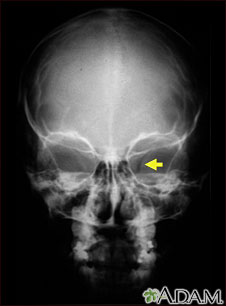The image is a digital screenshot of a frontal x-ray of a human head against a black background. The x-ray prominently features the outline of the eye sockets, jaw, and teeth. A short yellow arrow is pointing to the inside of the right eye socket. There is a white line originating from the top of the ears and curving around to the middle of the nose area, with a similar white line running down the center of the top part of the skull. At the bottom of the image, the name "Adam" is displayed alongside a green figure resembling a leaf or a palm tree. The main colors in the image are black, white, gray, yellow, and green.